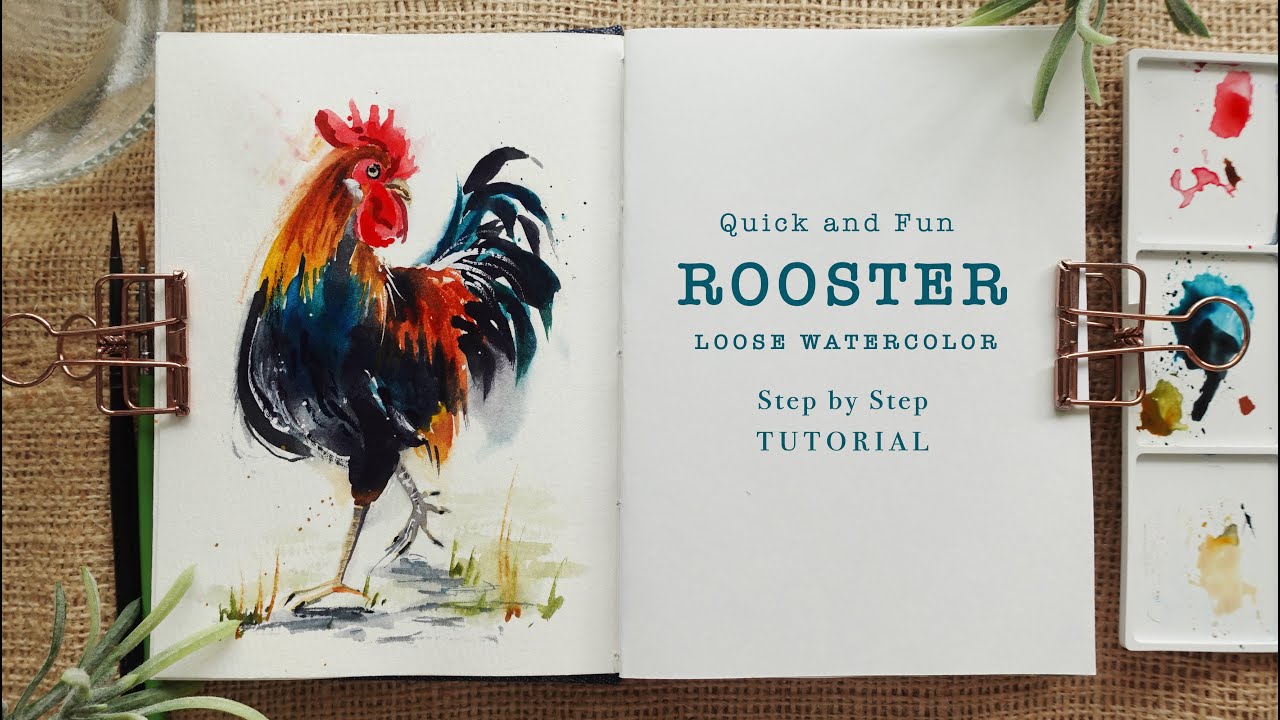In the image, there is an opened book clipped at both sides with simple metal clips, possibly repurposed from bag closures. The book is resting on a textured burlap fabric, providing a rustic backdrop. The left page displays a vibrant watercolor painting of a rooster, adorned with a vivid array of colors: a bright blue for the feathers, and a striking combination of red, orange, and yellow for the head and neck, complemented by strong gray legs. The rooster appears to be walking, with some grass depicted beneath it. Adjacent to this colorful illustration on the right page, the book cover reads "Quick and Fun Rooster Loose Watercolor Step-by-Step Tutorial" in blue font against a plain white background. Nestled to the left of the book are two tiny paintbrushes and part of a leafy plant, adding an artistic touch to the scene. On the right side, a paint tray with three compartments showcases splashes of red, blue, and yellow watercolors, enhancing the creative ambiance of the setting.